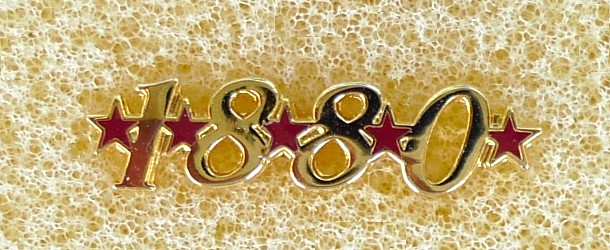The image features the number "1880" prominently displayed in shiny, reflective gold, with a slightly italicized font giving it a rightward slant. Each digit is separated by a red star with a gold outline, and additional red stars with gold outlines are placed before the '1' and after the final '0'. The background is a textured mix of white and cream-colored, bubble-like patterns that give the impression of cells under a microscope, with a heavier concentration of gold behind the numbers. The entire piece is set within a rectangular frame, presenting a harmonious blend of ornate detailing and vibrant colors, making it a unique piece of art.